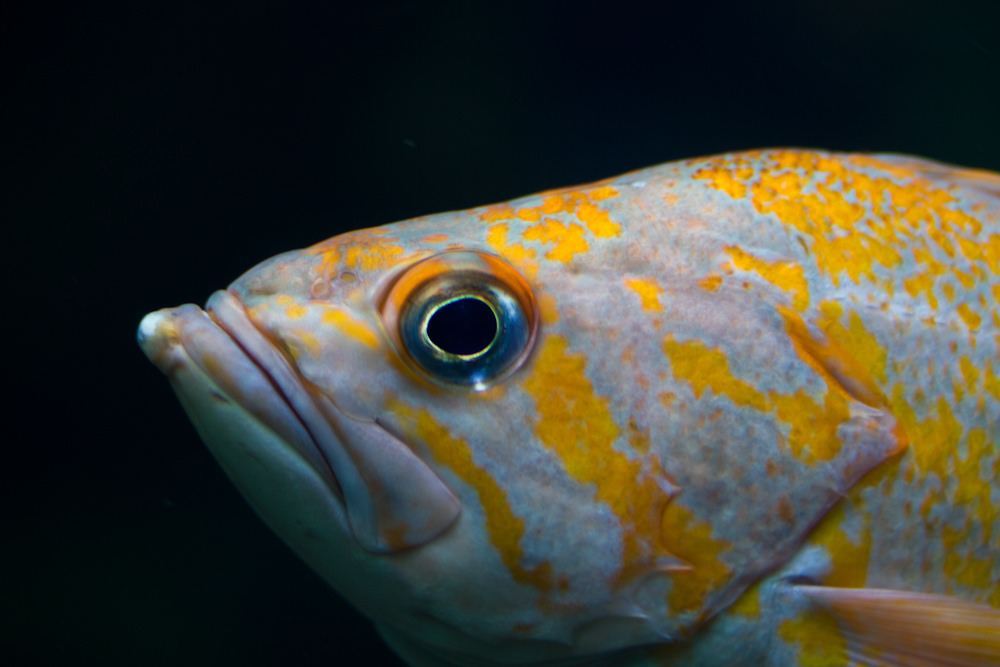The image features a close-up view of a fish's head and partial body set against a completely black background. The fish occupies the lower two-thirds of the frame, facing left, with its silvery eye and black pupil near the center of the composition. The mouth is closed, and the visible right-side fin is highlighted in pink. The fish's body showcases a splotchy pattern of bright yellow and gold spots and lines, set against a base color that varies between pinkish, bluish, and grayish tones. The head and gill area are prominently visible, while most of the body extends slightly beyond the frame. The fish's unique coloration, including its yellow speckles and stripes, creates a vivid contrast against the dark backdrop, making the details of its vibrant, multi-colored scales and fin stand out even more.